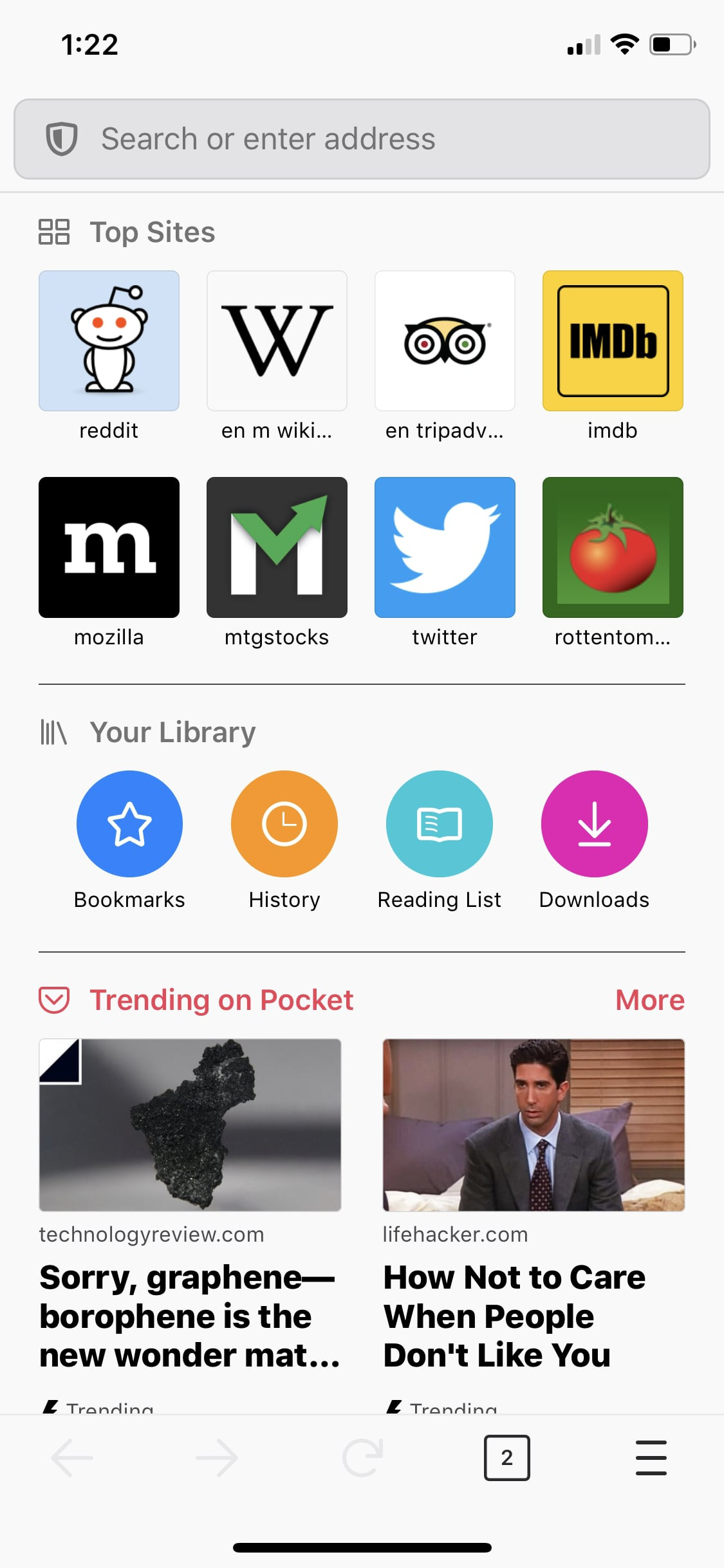At the top of the image, there is a status bar displaying "122" along with icons indicating that the Wi-Fi signal strength is at 2 out of 4 bars, and the battery is about half full. Below the status bar is a search bar with the prompt "Search or enter address." 

Underneath the search bar, a "Top Sites" section is visible, featuring icons and links to popular websites: Reddit, Wikipedia, TripAdvisor, IMDB, Mozilla, MTG Stocks, Twitter, and Rotten Tomatoes. 

A horizontal line separates this section from the next, which lists "Your Library" options: Bookmarks, History, Reading Lists, and Downloads. 

Another horizontal line beneath leads to two columns: on the left, it reads "Trending on Pocket," and on the right, it says "More." 

Below this, a highlighted article title on the left reads, "Sorry Graphene, Borophene, it's the new wonder MAT...," followed by another topic, "How Not to Care When People Don’t Like You."